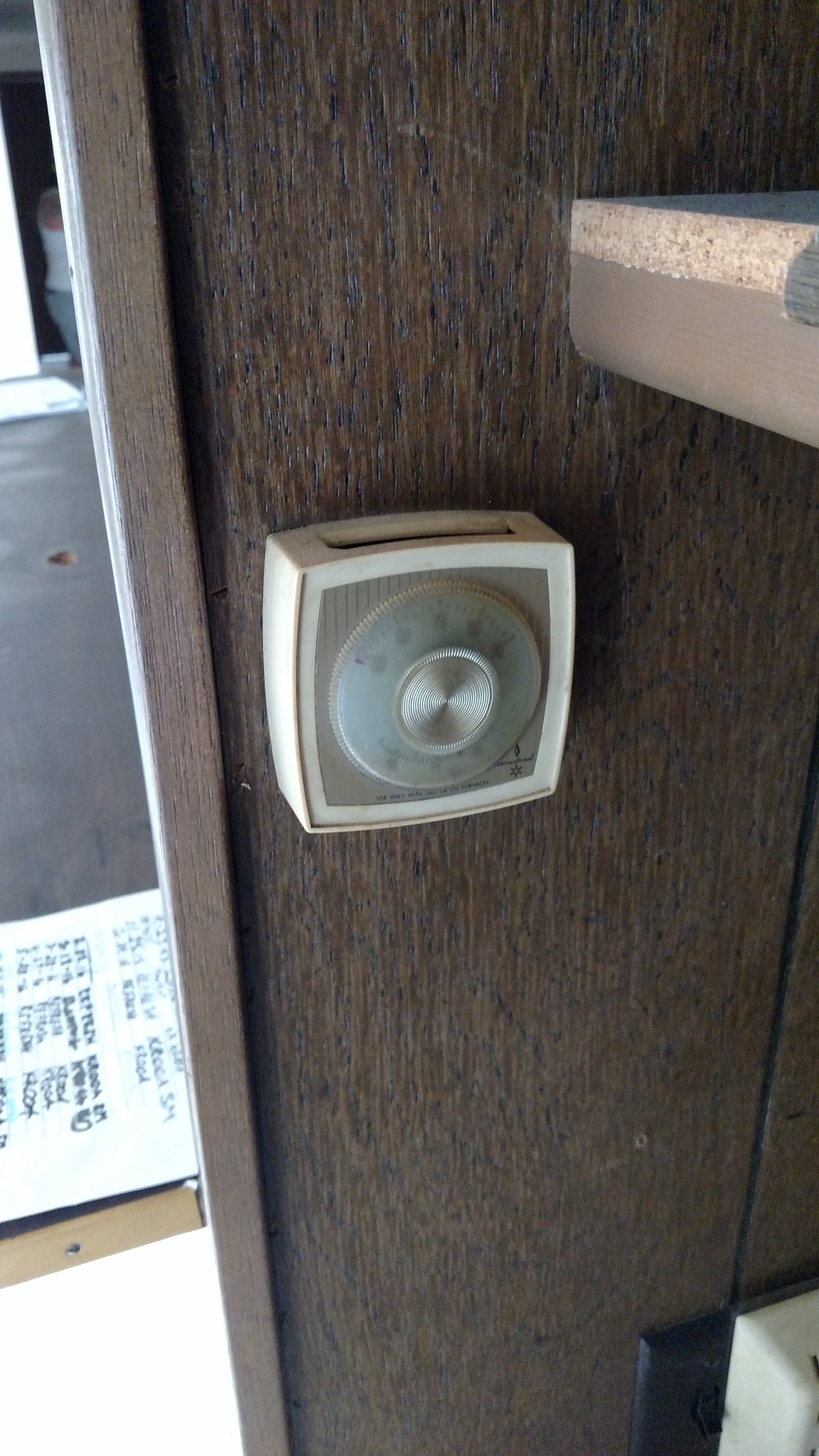The photograph, displayed in portrait orientation, captures a detailed interior scene dominated by a dark brown, paneled wood wall. The wall features a prominent black seam running upwards. Centrally located on the wall is an older, white plastic-encased thermostat with a dial, not digital, featuring numbers and a mysterious slot at the top hinting it could be something other than a thermostat.

Below the thermostat, a black plate covers an electrical outlet into which a white plastic object is plugged. Above the thermostat hangs a silver shelf, which appears to be wooden. 

To the right, the frame extends to include part of a door frame beyond which a very bright light spills into the room. Near this doorway is a gray metal object adorned with small blue patterns, brightly lit toward its base, suggesting an internal light source. This metal object sits atop a small wooden shelf. In the distance, the room contains additional, indistinct objects.